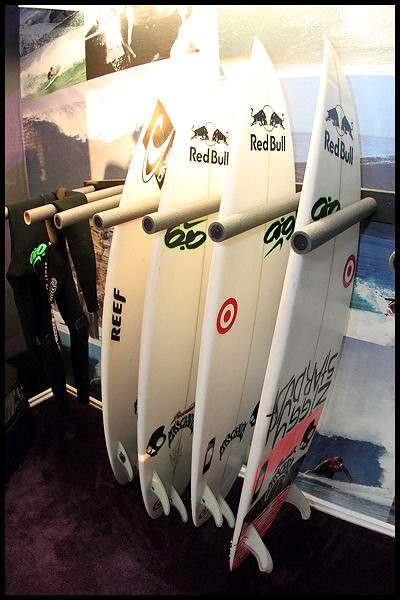The image depicts a detailed scene of a surfboard display, possibly in a surf shop or a private surfboard room. There are four surfboards neatly stored in a rack, where the rack consists of silver cylindrical bars that hold the boards upright against a mostly white wall with blue elements. Each surfboard is predominantly white with distinct branding and artwork:

1. **Leftmost Surfboard:** It carries the "Reef" logo in black text.
2. **Second Surfboard:** Features the iconic Red Bull logo along with a red and white Target symbol.
3. **Third Surfboard:** Also branded with Red Bull and bears a Target symbol, plus it reveals the name "Ziggy Stardust" written upside down.
4. **Rightmost Surfboard:** Similarly marked with the Red Bull logo and Target emblem.

In addition, there is some surfer gear hanging on the front two bars of the rack, with colors including black, white, and green. The floor beneath the rack is a dark purple, almost black, providing a rich contrast to the white surfboards. The surrounding wall is decorated with tiles displaying surfing scenes—from waves to surfers in action—further enhancing the theme of the space. The photograph, framed by a medium-thick black border, ensures the surfboards remain the central focus of this colorful and vibrant display.